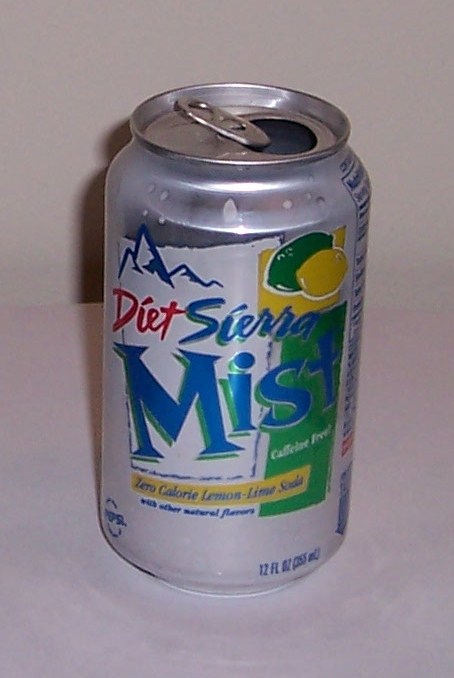This is an up-close digital photograph of a silver Diet Sierra Mist soda can set on a hard surface, likely a table, against a beige or white indoor background. The background features a grey wall and casts a shadow behind the can, creating a slight separation indicating the table surface. The can has an open pop-top in an upright position, with the opening visible. The can's label includes a prominent white square in the center. In the upper part of the square, outlined in blue, there's a depiction of steep mountain peaks. Below this, the word "Diet" is written in red cursive text, to the right of which "Sierra" appears in blue cursive text, and beneath is the word "Mist" in regular print. In the upper right corner of the label is a yellow square containing images of a lime and a lemon. Below this square, the background transitions to a light green shade. Across the bottom of the white square is a yellow rectangle with blue writing that reads "Zero Calorie Lemon Lime Soda." Additionally, towards the bottom of the can, the word "Pepsi" is in blue text on the left, and "12 FLOZ (355 ML)" is on the right. The can also carries the phrase "Caffeine Free" in white lettering.